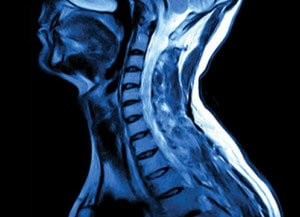This image presents an intricately detailed x-ray-like illustration of a person's throat and neck area, rendered in shades of blue, white, and black. The skeletal structure, including the vertebrae, mandible, and curvature of the spine, is prominently displayed against a completely black background. This side-profile view captures not only the skeletal framework but also suggests muscle tissue with darker tones and bone structures in brighter whites. While it resembles a traditional medical x-ray with transparent qualities, there is an artistic element to the imagery that makes it appear more like a stylized, frosted acrylic or plastic model potentially used for teaching purposes. The depiction extends to include the base of the brain and the medulla, further enhancing its medical accuracy and depth.